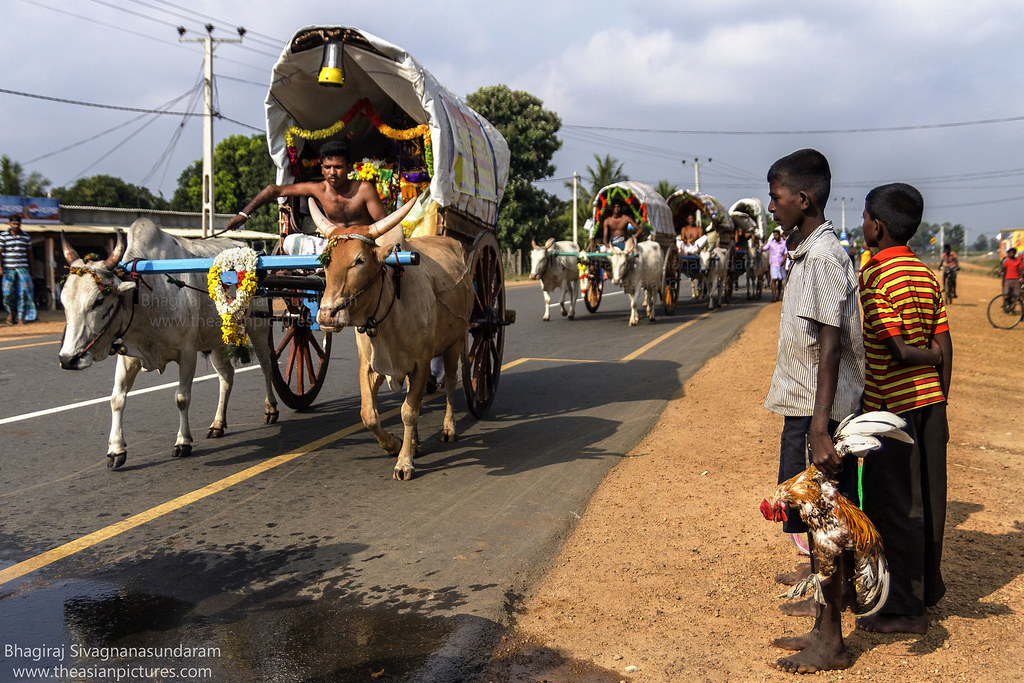This photograph captures a vibrant parade-style procession making its way down a road. The scene could be a ceremony, a funeral, or perhaps a traditional parade. Lining the road, spectators watch attentively, adding to the sense of community and occasion. In the foreground, two boys stand close to the camera; one of them is holding a dead chicken, adding a curious detail to the event. The procession features numerous wagons, all adorned with colorful decorations and flowers, showcasing intricate details that add festive flair. Each wagon is pulled by long-horned cows, which are integral to the procession and contribute to the cultural richness of the scene.